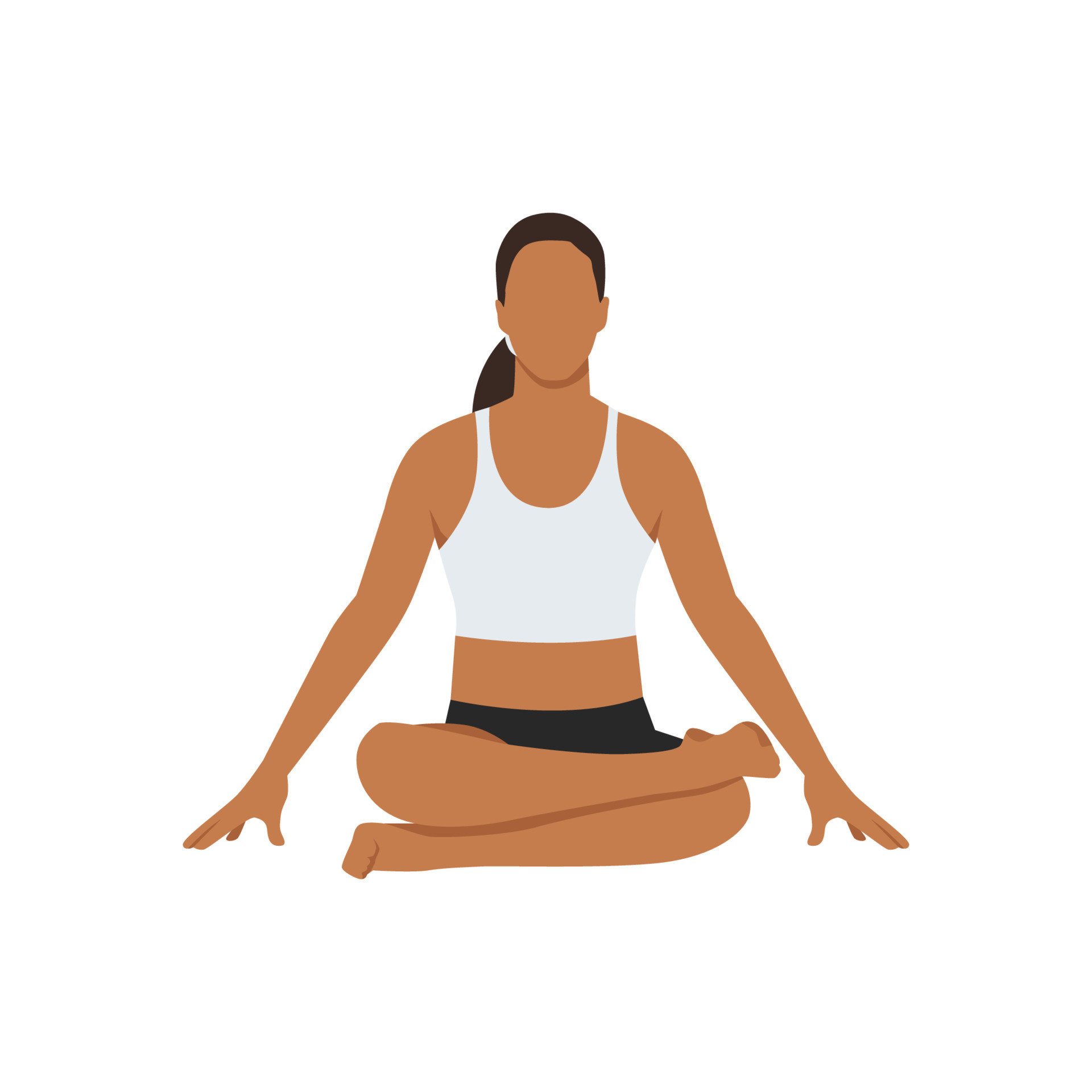The illustration depicts a simplistic, computer-generated image of a woman in a yoga pose, set against a pristine white background. She is seated cross-legged, with her right leg draped over her left. The woman has slightly dark skin, a very light brown shade, and is dressed in dark pants or shorts visible only slightly above the waist, along with a white sports bra that shows her midriff. Her arms are extended to the sides, with her fingertips gently touching the ground. She has dark, thin hair pulled back into a ponytail that drapes over her left shoulder. Notably, her face lacks any features, adding to the minimalistic style of the artwork. Overall, the image is characterized by its simplicity and peaceful composition.